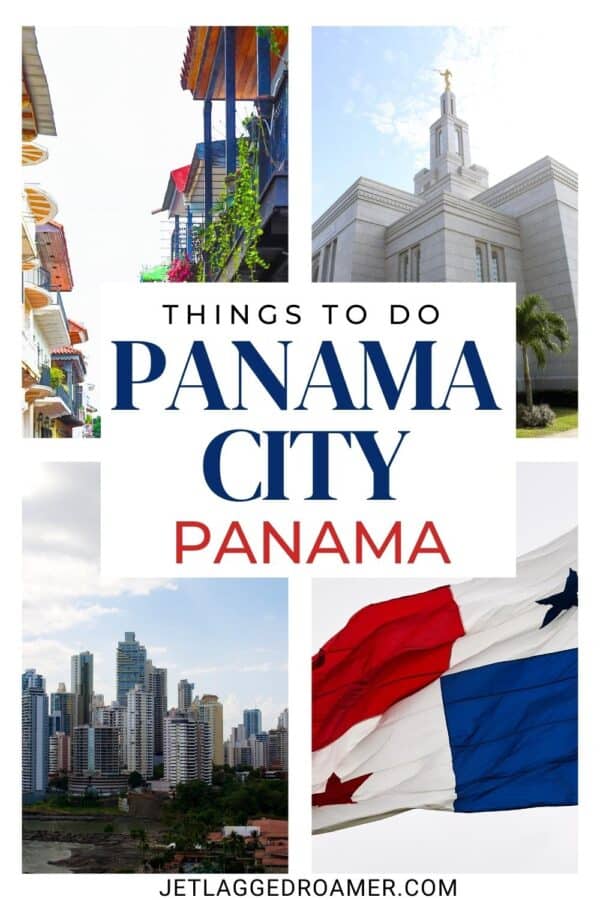The image is a neatly arranged collage showcasing various scenes from Panama City, Panama. In the center, bold black text reads "things to do," followed by "Panama City" in large blue font, and "Panama" in striking red font, all set against a clean white square background. At the bottom, the text "jetlaggedroamer.com" is clearly visible.

The collage consists of four distinct images: 

1. The top-left corner features a street view with taller buildings. Though partially obscured by the central text, visible elements include overhanging, covered patios—one notably blue with greenery trailing over its railing.
 
2. The top-right corner displays a white building, possibly a church, characterized by its elegant architecture and apparent steeple.

3. The bottom-left image captures a dynamic city skyline filled with towering buildings and skyscrapers, highlighting the urban aspect of Panama City.

4. The bottom-right image showcases the national flag of Panama waving gracefully in the wind.

This collage serves as a vibrant visual guide to the architectural and cultural highlights of Panama City, enticing viewers with its diverse attractions.